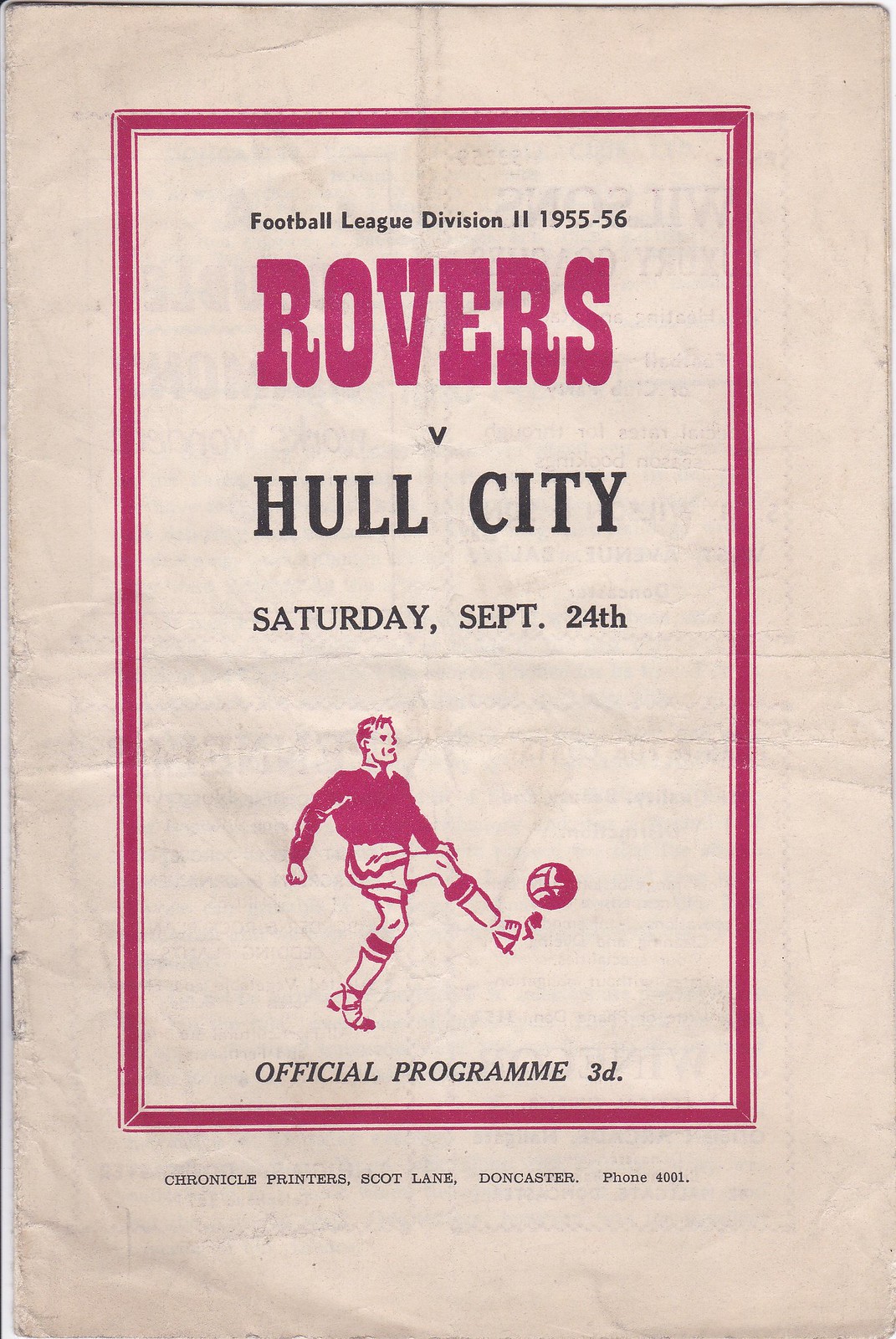This image showcases an official football program from the Football League Division 2 match between Rovers and Hull City, held on Saturday, September 24, 1955. The program, designed in a vintage pink and white color scheme, features the title "Football League Division 2 1955-56" prominently across the top. Beneath the title, the matchup "Rovers vs. Hull City" and the date are clearly stated. The cover includes a simplistic yet eye-catching illustration of a footballer, dressed in a sweatshirt, shorts, knee socks, and cleats, actively kicking a soccer ball. Below this illustration, it reads "Official Program 3D," indicating the price. Further down, the printer's details are specified as Chronicle Printers, Scott Lane, Doncaster, with the phone number 4001. The program shows visible signs of aging, such as wrinkles, which add to its historic charm.